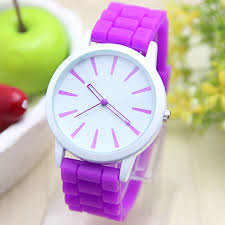A detailed close-up photograph captures an analog watch with a distinctive, minimalist design. The watch's face is white and circular, displaying only purple lines in place of numerical indicators. The hour, minute, and second hands are also purple, matching the minimalist aesthetic. The band of the watch appears to be made of a purple silicone or rubber material, featuring a quilted design that adds texture and visual interest.

In the background to the left, there is an indistinct, blurry green apple situated inside what seems to be a white tub or bowl. Adjacent to the apple is a mysterious red object, partially obscured and undefined. Further in the background, there is another blurred object with hues of green and yellow, though its exact nature is indiscernible due to the focus on the watch. The watch itself is resting on a surface that resembles white marble, enhancing the clean, sophisticated presentation of the timepiece. There are no text elements or additional context provided in the image.